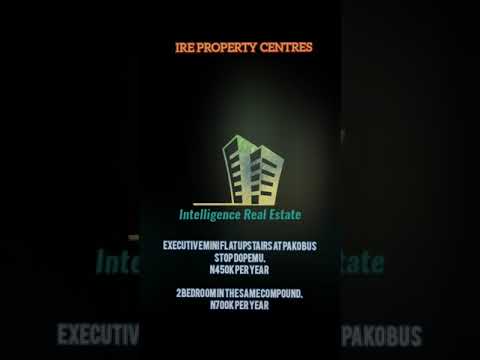The image appears to be an advertisement from a magazine, with a sleek black background accentuated by white or grey highlights as if illuminated by a spotlight. Dominating the top and center of the page is the text "IRE (Intelligence Real Estate) Property Centres" in red. Below this, a stylized illustration features two skyscrapers, one slightly leaning to the left and the other to the right. The tagline "Intelligence Real Estate" is displayed in blue beneath the skyscrapers. Further down, in white text, it reads "Executive Mini Flat Upstairs at Pacobus. Stop Dopimu. N450K per year, two-bedroom in the same compound N700K per year." A watermark appears in the lower-left corner, with partially legible text reading something akin to "EXECUTE TIV" and "PACKOBOS."